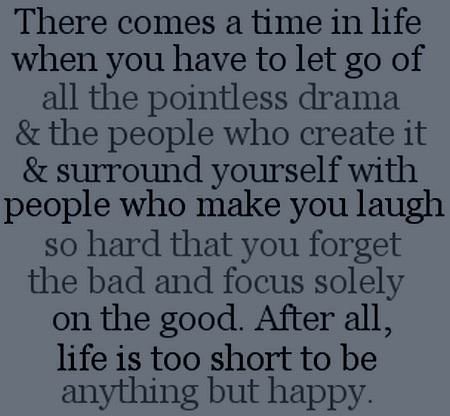The image displays a simple square with sides of equal length against a solid dark gray background. Within the square, multiple lines of text are arranged from top to bottom, conveying a poignant message. The text reads: "There comes a time in life when you have to let go of all the pointless drama and the people who create it and surround yourself with people who make you laugh so hard that you forget the bad and focus solely on the good. After all, life is too short to be anything but happy." The text alternates between black and a slightly darker gray, adding a subtle variation within the uniform grid. The contrast between the dark gray background and the alternating shades of text highlights the powerful message about prioritizing happiness and positivity in life.